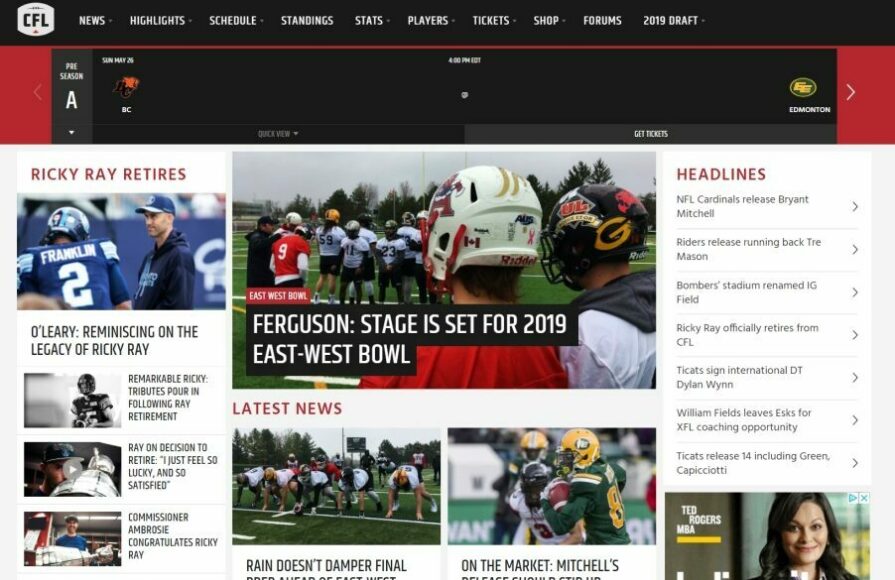**Caption: Comprehensive CFL Web Page Overview**

The web page is dedicated to the Canadian Football League (CFL) and features various sections such as News, Highlights, Schedule, Standings, Stats, Players, Tickets, Shops, Forums, and the 2019 Draft. The page is currently focused on the preseason, with a specific emphasis on Sunday, May 26, detailed under a dropdown marked by the letter "A". The event highlights a game between BC and Edmonton, indicated by an unfamiliar icon next to BC and two "E"s enclosed in a circle next to Edmonton. This game is scheduled to start at 4:00 PM Eastern Standard Time.

On the left-hand side, there is a "Quick View" section, although the "Get Tickets" view is currently highlighted. The page is filled with numerous images and headlines. One notable section highlights Ricky Ray's retirement with multiple articles such as "Ricky Ray Retires," "O'Leary Reminiscing on the Legacy of Ricky Ray," accompanied by a picture of a coach and a football player. Another article titled "Remarkable Ricky: Tributes Pour In Following Ray Ray Retirement" is displayed next to a picture of the football player. Ricky Ray's personal reflections are captured in the headline "Ray on the Decision to Retire: 'I Just Feel So Lucky and So Satisfied'," accompanied by a video of someone kissing a trophy. A still image of a man holding a trophy is linked to an article titled "Commissioner Ambrose Congratulates Ricky Ray."

In the center, the section highlights the East-West Bowl with the headline "East-West Bowl Ferguson: Stage is Set for 2019 East-West Bowl," showing several images of people playing football. 

Underneath, there is a section titled "Latest News" in red text, which includes an article "Rain Doesn't Damper Final," showing players huddled on the line. There's a partially visible headline starting with "On the market, Mitchell's," associated with a team in green and yellow uniforms.

On the right-hand side, the "Headlines" section features numerous news items, each indicated with a greater-than sign for more details:
- "NFL Cardinals Release Bryant Mitchell"
- "Riders Release Running Back Trey Mason"
- "Bomber Stadium Renamed IG Field"
- "Ricky Ray Officially Retires from CFL"
- "Thai Cat Sign International DT Dylan Nguyen"
- "Williams Field Leaves Esks for XFL Coaching Opportunity"
- "Thai Cats Release 14, including Green and Capiciotti"

Additionally, there is a mention of "Ted Rogers NBA" with a picture of a woman beside a blue triangle and blue X.

The page presents a thorough representation of recent CFL events, prominent retirements, and the latest league news, enriched with images and engaging headlines.